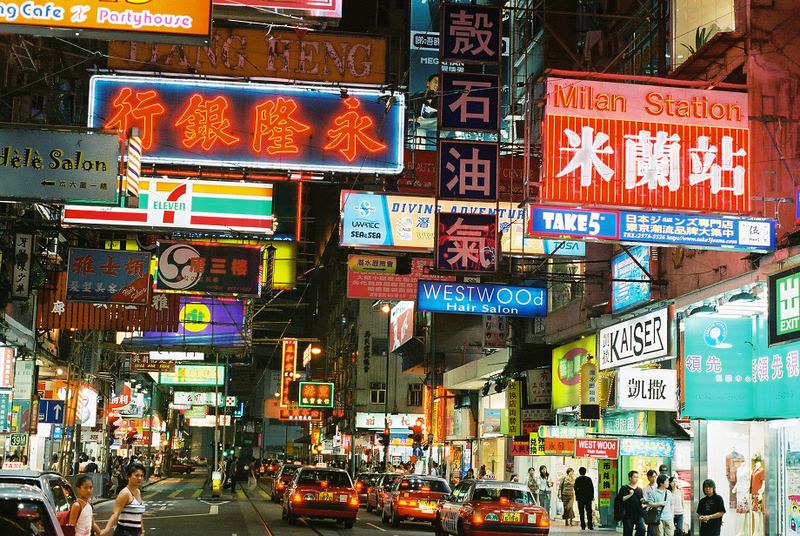The photograph captures a bustling Asian city street at night, illuminated with a plethora of fluorescent lights that fill the scene and obscure the sky. The road is crowded with several vehicles, their brake lights glowing, as two people attempt to cross the street. On both sides of the road, vibrant shop buildings with well-lit signs and banners advertise various products. These signs are densely packed together, displaying text in both Chinese and English languages, with notable mentions such as "7-Eleven," "Milan Station," and "Westwood Hair Salon." The brightly lit advertisements and storefronts contribute to a lively atmosphere, typical of a busy downtown area. Pedestrians are seen walking and window shopping on the crowded sidewalks, emphasizing the street's energetic vibe. The overall scene evokes a hectic yet vibrant Chinatown-like setting.